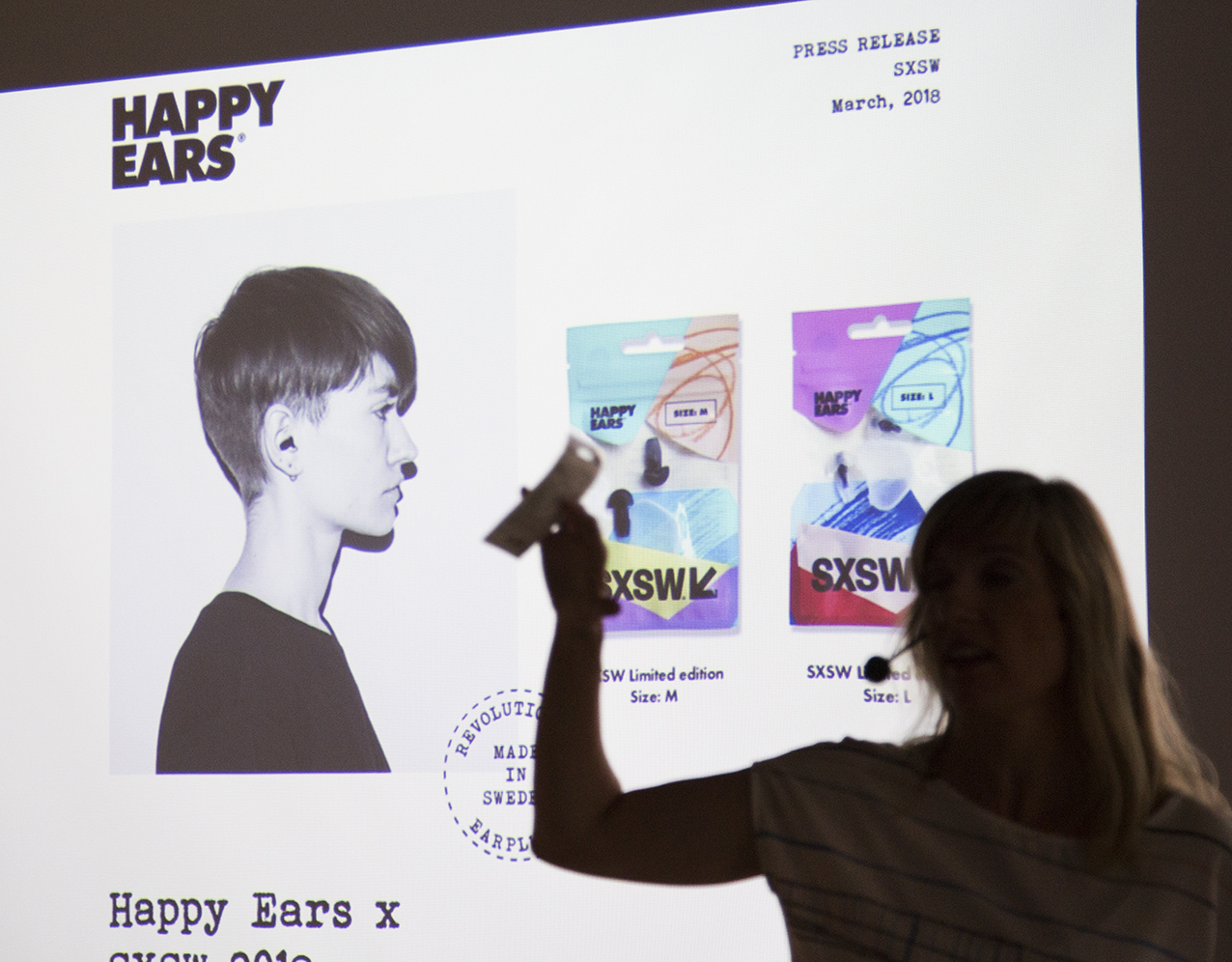In this image, we see a woman positioned in the bottom right corner, facing the camera, with a headset microphone attached to her left ear. She has long hair and appears to be holding a piece of paper in one hand, raising it slightly as she speaks into the microphone. The woman is in shadow, adding to the dark ambiance of the scene, which appears to be set in a dimly lit indoor room.

Behind her, there is a projected screen displaying the text: "Happy Ears Press Release SXSW March 2018." The projection also includes images of a boy with short dark hair and earrings, along with several products next to him, which look like earplugs or earbuds. Additional text on the screen reads: "Limited Edition Size M," "SXSW Limited Edition Size L," "Revolutionary," "Made in Sweden," and "Ear Plugs Happy Ears X."

The image features a blackish background, and the colors visible include black, white, different shades of gray, light blue, orange, tan, blue, purple, and red. The boy and the earplugs are centrally positioned in the projection, emphasizing their importance in the presentation.